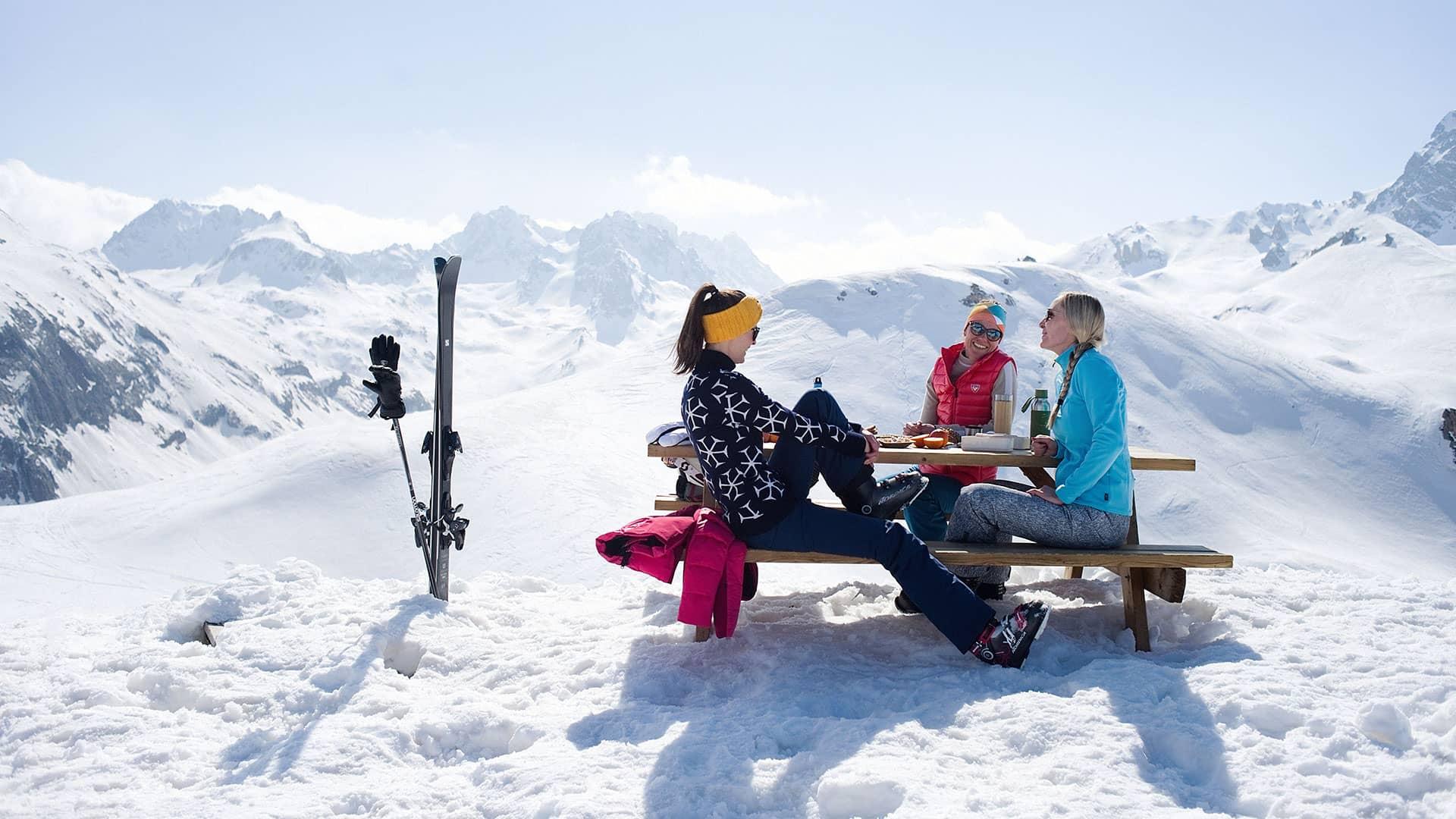In this landscape photo, three women are casually seated at a wooden picnic table on a snowy mountaintop, under a crisp blue sky with scattered clouds. Surrounding them are the steep, snow-covered peaks of the mountains, creating a stunning, wintry backdrop. Skis, poles with gloves atop, are planted vertically in the deep snow on the left side of the image.

The woman on the left sits with her left knee drawn to her chest, dressed in a black coat adorned with white snowflakes, blue pants, and ski boots, all complemented by a yellow headband. She sits atop a pink coat. To her right, a blonde woman faces inward, wearing a light blue jacket, gray pants, and sunglasses, typical for a ski trip. The third woman, positioned at the far side of the table, looks at the blonde. She is sporting a red puffer jacket, an orange and blue hat, sunglasses, and sits comfortably involved in their group dynamic. Each woman is layered in appropriate winter attire, prepared for the snowy setting.

On the wooden table in front of them sit a green water bottle, a brown water bottle, and a piece of fruit, suggesting they are enjoying a meal after skiing. The vibrant colors of their outfits and the gear contrast sharply against the pristine white of the snow and the expansive, azure sky, capturing a moment of leisure and camaraderie in an idyllic, alpine environment.